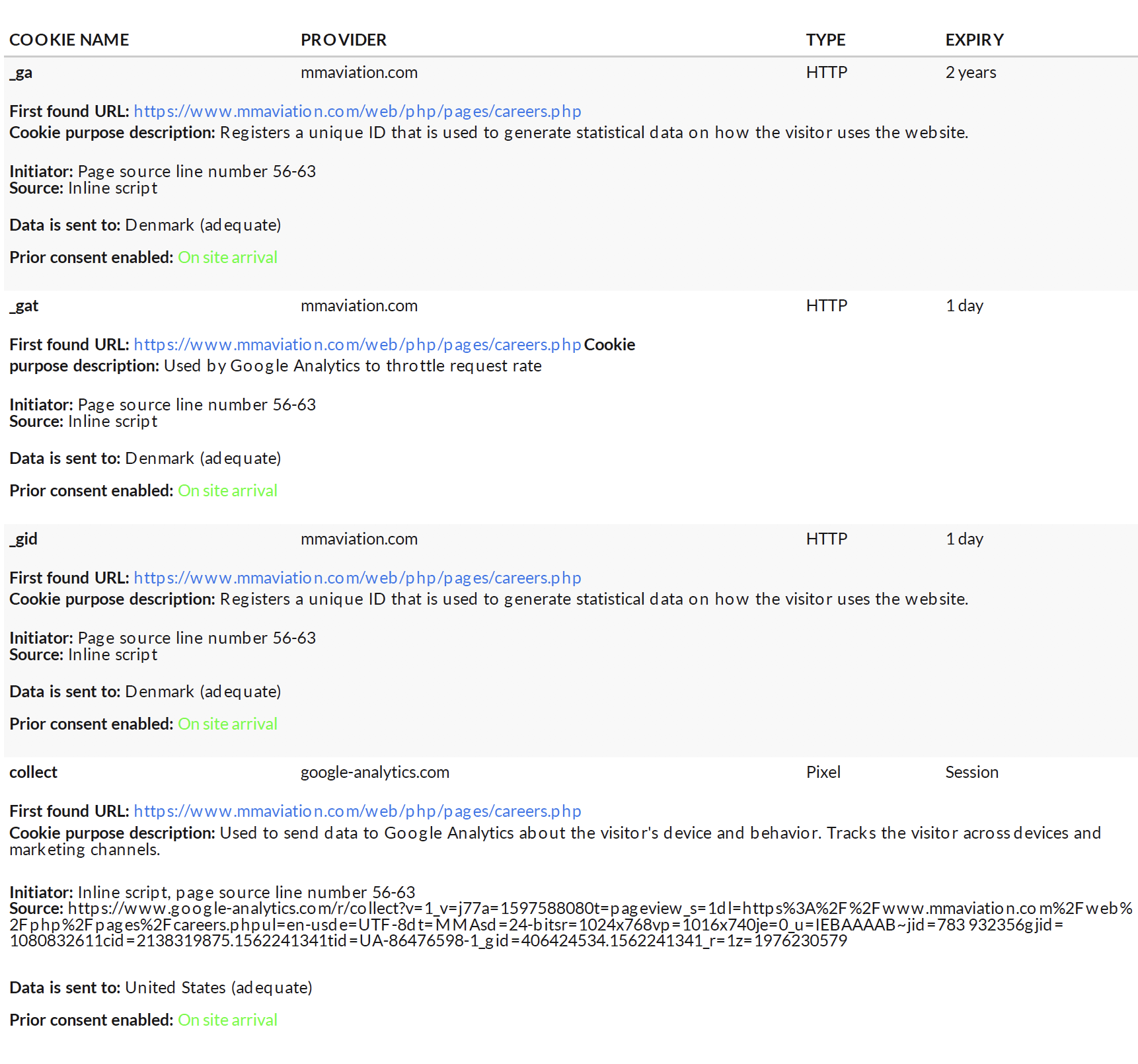This image shows a detailed table describing various cookies used on the mmaviation.com website. Each cookie entry provides comprehensive information, including the cookie name, provider, type, and expiry date. Here's a breakdown:

1. **Cookie Name:** _ga
   - **Provider:** mmaviation.com
   - **Type:** HTTP
   - **Expiry Date:** 2 years
   - **Data Sent To:** Denmark
   - **Prior Consent Enabled:** On-site arrival (green)

2. **Cookie Name:** _gat
   - **Provider:** mmaviation.com
   - **Type:** HTTP
   - **Expiry Date:** 1 day
   - **Data Sent To:** Denmark
   - **Prior Consent Enabled:** On-site arrival (green)

3. **Cookie Name:** _gid
   - **Provider:** mmaviation.com
   - **Type:** HTTP
   - **Expiry Date:** 1 day
   - **Data Sent To:** Denmark
   - **Prior Consent Enabled:** On-site arrival (green)

4. **Cookie Name:** collect
   - **Provider:** Google Analytics
   - **Type:** Pixel
   - **Expiry Date:** Session
   - **Data Sent To:** United States
   - **Prior Consent Enabled:** On-site arrival (green)

The table further includes additional data points like the first found URL, cookie purpose description, initiator, and source. These details provide transparency on how user data is handled and where it is sent.